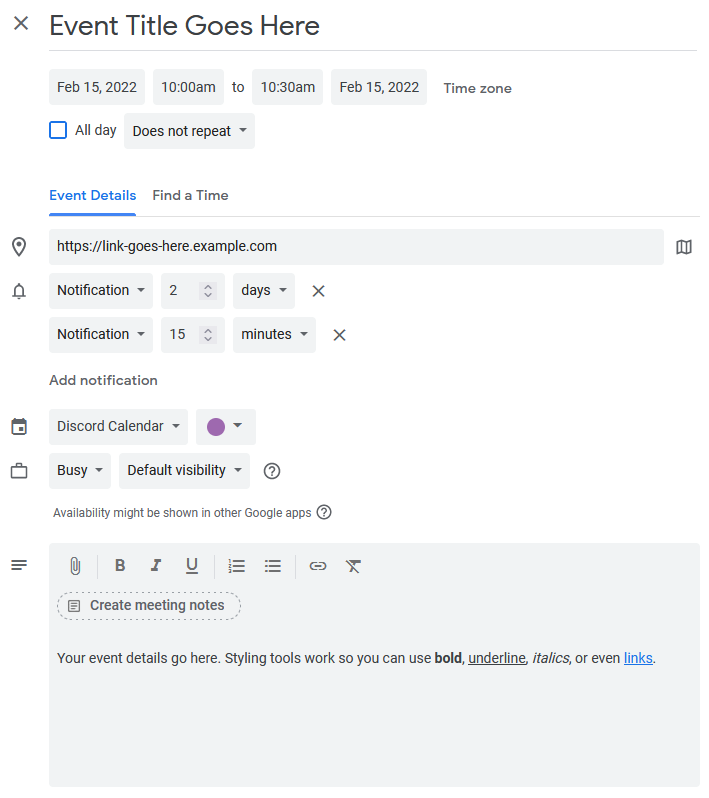The image depicts a Google Calendar event creation page with a predominantly white background. At the top of the window, a close (X) icon is flanked by the text "Event title goes here" in black, underlined by a horizontal line. Below, the interface allows setting the event's start and end dates and times, which are February 15th, 2022, from 10:00 AM to 10:30 AM. There is also an option to select the time zone. A small checkbox labeled "All day" can be toggled, and a drop-down menu shows "Does not repeat" for event recurrence.

Further down, two options, "Event details" and "Find a time," are displayed side by side. "Event details" is highlighted in blue, indicating it is selected. Directly under this, a location icon (pin drop) is visible next to a text box for entering the event's location. Below the location input, a notification icon is present, allowing the user to set reminders for the event. The event is currently set to be added to a "Discord" calendar. There is also an option to select the alert color, which is shown as purple. Lastly, users can choose the visibility status of the event as well as whether they want to appear busy or free.

At the bottom of the screen, a gray text box provides space for additional comments or details, with options to format the text in different styles.